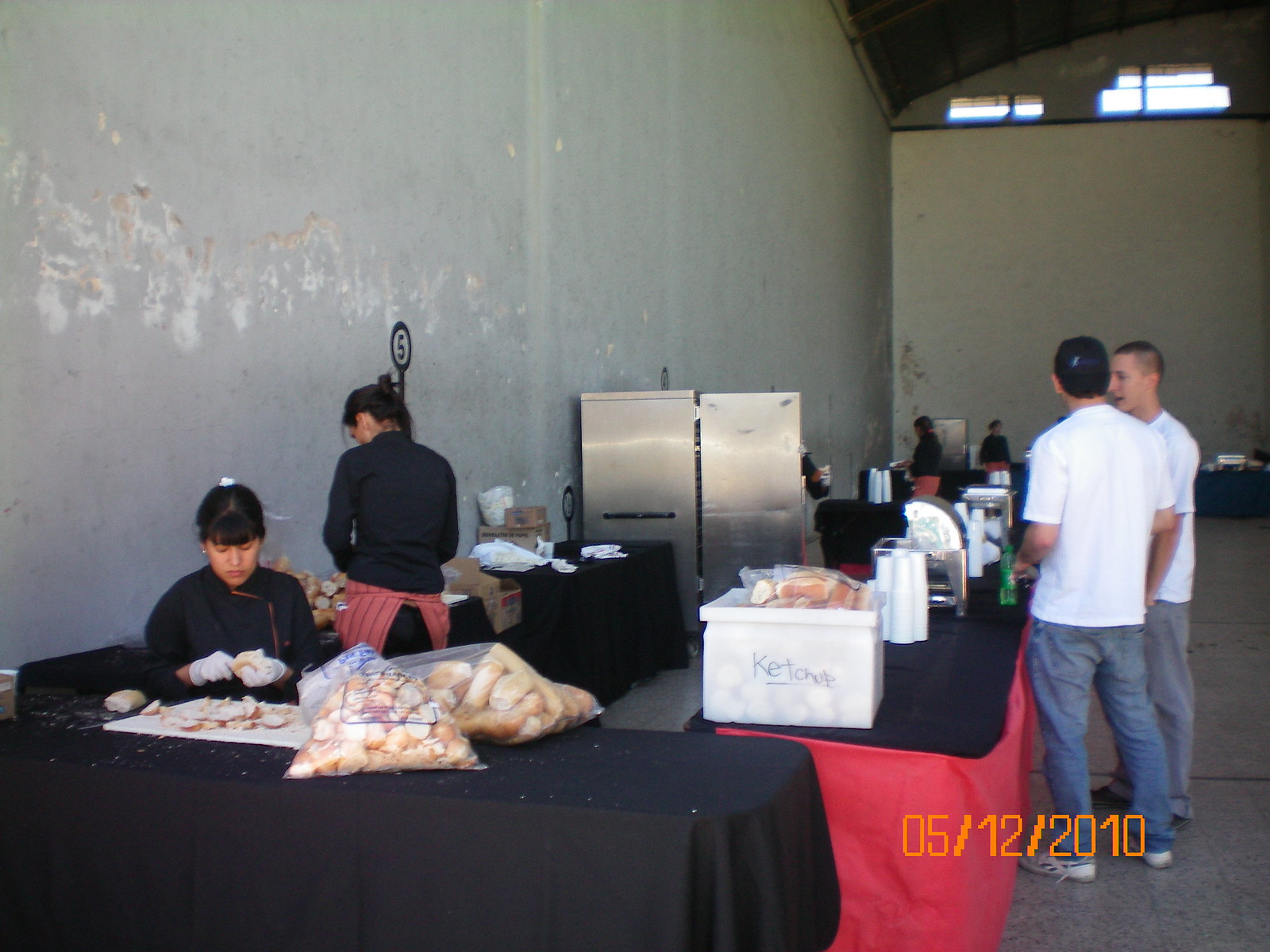The photograph, dated May 12, 2010, captures a bustling scene in a large concrete warehouse, set up like a catering or food prep station. The setting features three tables staffed by two women in black chef uniforms, who appear to be cutting food items such as potatoes, onions, or bread. Notably, there’s a box labeled "ketchup," although it contains loaves of bread. At the right side of the tables, two men dressed in white shirts and blue jeans are engaged in a conversation. Further in the background, more people and tables are visible, suggesting a larger-scale operation. Against the wall at the end of the row of tables is a refrigerator with its door open; a person's figure is mostly obscured by the door. A notable detail on the wall is a number five within a circle, the significance of which is unclear. The entire scene takes place on concrete floors within the warehouse, and the timestamp on the bottom right of the photograph reads 05/12/2010 in orange.